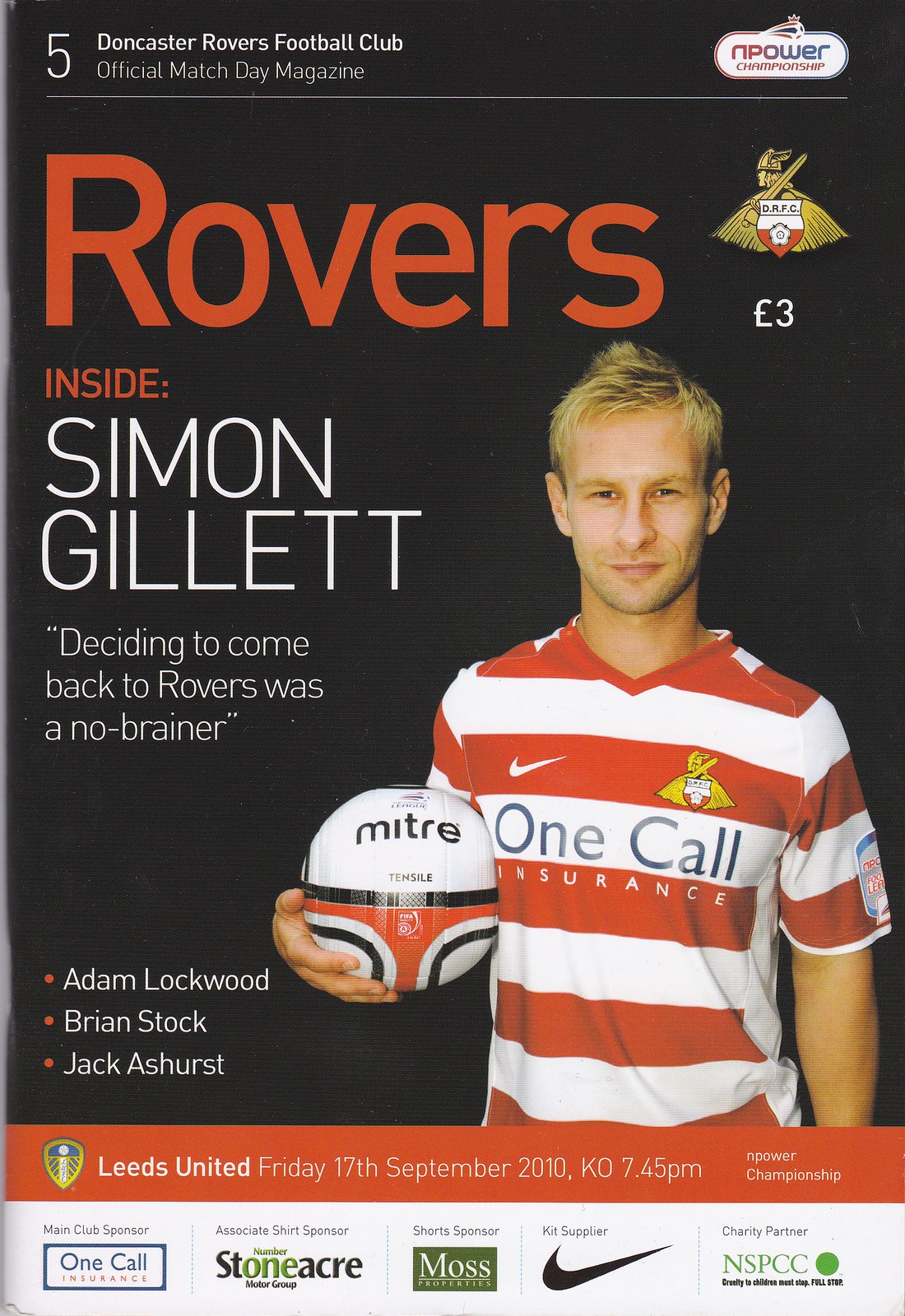This detailed caption describes the magazine cover thoroughly:

The image features the cover of the "Doncaster Rovers Football Club Official Match Day Magazine". The background at the top is black with "Rovers" prominently displayed in large red letters. To the right of this title is a logo, likely for the N-Power Championship, with text in white and red. Underneath, it reads "Inside: Simon Gillette" followed by a quote in white capital letters: "Deciding to come back to Rovers was a no-brainer."

In the upper left-hand corner, the number 5 is visible. A team logo and the price of the magazine, three pounds, are also present near the top. The cover predominantly features a color photograph of a blonde man, presumably Simon Gillette, holding a soccer ball in his right arm while wearing a red and white striped jersey with the text "One Call Insurance" on it and a Nike swoosh over the left side.

At the bottom left of the cover, three names are listed in white: Adam Lockwood, Brian Stock, and Jack Ashurst. A red banner stretches across the bottom of the page with details in white about an upcoming match: "Leeds United, Friday 17th September 2010, K.O. 7:45 PM". Below this, in white text, are several logos and symbols indicating sponsors and partners including One Call Insurance, Stoneacre, Moss, Nike, and NSPCC.